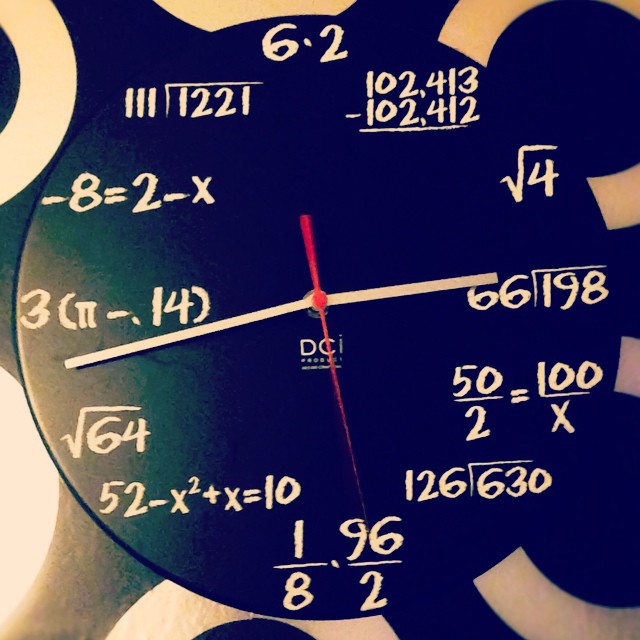This color photograph captures a unique decorative piece placed on a solid surface, composed of a black circular base with a beige top. The centerpiece of the image is a clock-shaped object featuring a black circular face with three hands: a red second hand, and two black hands for the hour and minute. The time indicated is 3:44 and 29 seconds. Instead of numerals, various mathematical problems are displayed around the clock face. These problems include equations such as '-8 = 2 - X,' 'Square root of 64,' and '630 divided by 126.' This piece blends the aesthetic of a traditional clock with the intellectual challenge of arithmetic, creating an intriguing and visually stimulating creation.